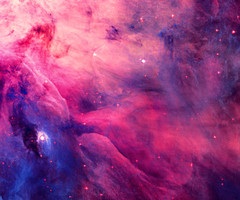This image is a highly detailed and abstract representation of a stellar phenomenon, possibly resembling a supernova. The scene appears almost computer-generated, presenting a vibrant spectacle typically seen in space photographs. Dominating the composition, clouds of pink smoke extend from the left side, sweeping across the image to the right. These clouds intermingle with spots that resemble stars, giving the picture a cosmic vibrance. 

On the lower left side, amidst the darker blue and black hues of the cloud cover, a bright, shiny white dot stands out, seemingly encased in a shrouding cloud. This bright spot, coupled with various tones of purple, pink, and light pink cloud formations across the image, creates a compelling and colorful celestial display. Particularly intriguing is the formation at the bottom left, which some might interpret as an eye or possibly the face of an animal, adding to the image's mystique and complexity. 

With stars scattered throughout and varied coloration blending seamlessly, the image captures the chaotic beauty of space, drawing viewers into a mesmerizing cosmic landscape.